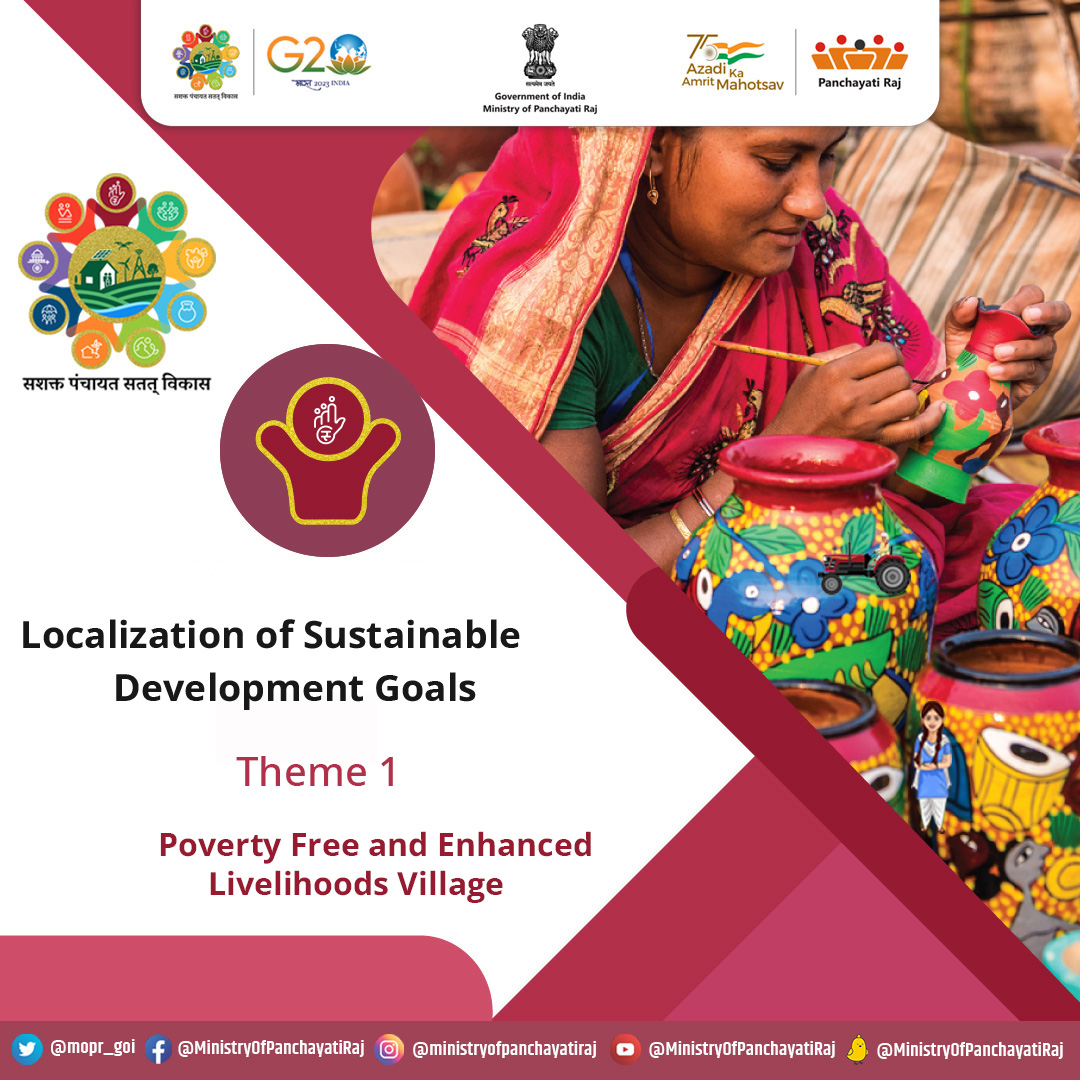This flyer or presentation title slide is divided diagonally, creating two triangular sections from the top left to the bottom right. At the top, there's a banner adorned with multiple logos, including the subtitle "Government of India, Ministry of Panchayati Raj" and additional logos for Panchayati Raj. The bottom banner features social media addresses for Twitter (@MOPR_GOI), Facebook, Instagram, YouTube, and a social web logo resembling a yellow duck.

The left triangle, with a white background and a red border separating it from the right section, hosts the text "Localization of Sustainable Development Goals. Theme 1: Poverty-Free and Enhanced Livelihoods Village." The right triangle contains a photograph of an Indian woman in traditional attire. She is dressed in a patterned bright reddish-pink sari with a head covering and a green shirt, and she has brown skin and a gold hoop earring. The woman is captured in the act of hand-painting flowers on pottery vases, with several of her completed works visible in front of her.